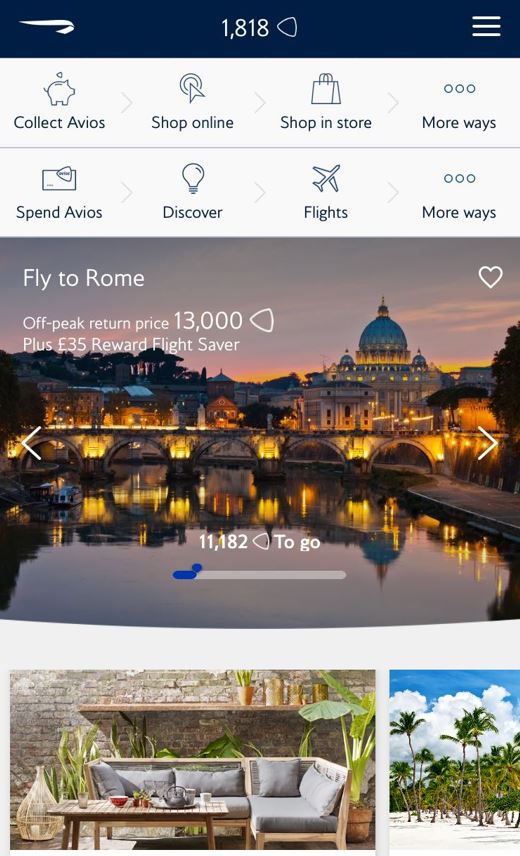**Screenshot Description: Travel Website Overview**

The screenshot features a travel website's main page. Prominent at the top is a dark blue navigation bar with a distinctive white swirl, though the website's name is not visible. Centered on this swirl, there's the number "1818" and an icon resembling a guitar pick. On the far right of the bar, a classic three-horizontal-line menu button is present.

Below this bar, the website's background is stark white, segmented into two rows of four options each. These options include:

- **Top Row:** 
  1. Collect Avios
  2. Shop Online
  3. Shop In Store
  4. More Ways

- **Second Row:**
  1. Spend Avios
  2. Discover
  3. Flights
  4. Another "More Ways" option

Dominating the center of the page is a high-resolution image of Rome, capturing a scenic view of a river with historic buildings and bridges, reminiscent of architectural marvels found in the city. In the top-left corner of this image is a promotional text stating: "Fly to Rome," advertising off-peak return prices at "13,000 Avios plus 35." The currency or points of the additional 35 were ambiguous, potentially being francs or euros, akin to a reward flight saver fee.

Overall, the website seems dedicated to travel and avios points management, offering various options for spending and collecting Avios, along with encouraging travel-related purchases.